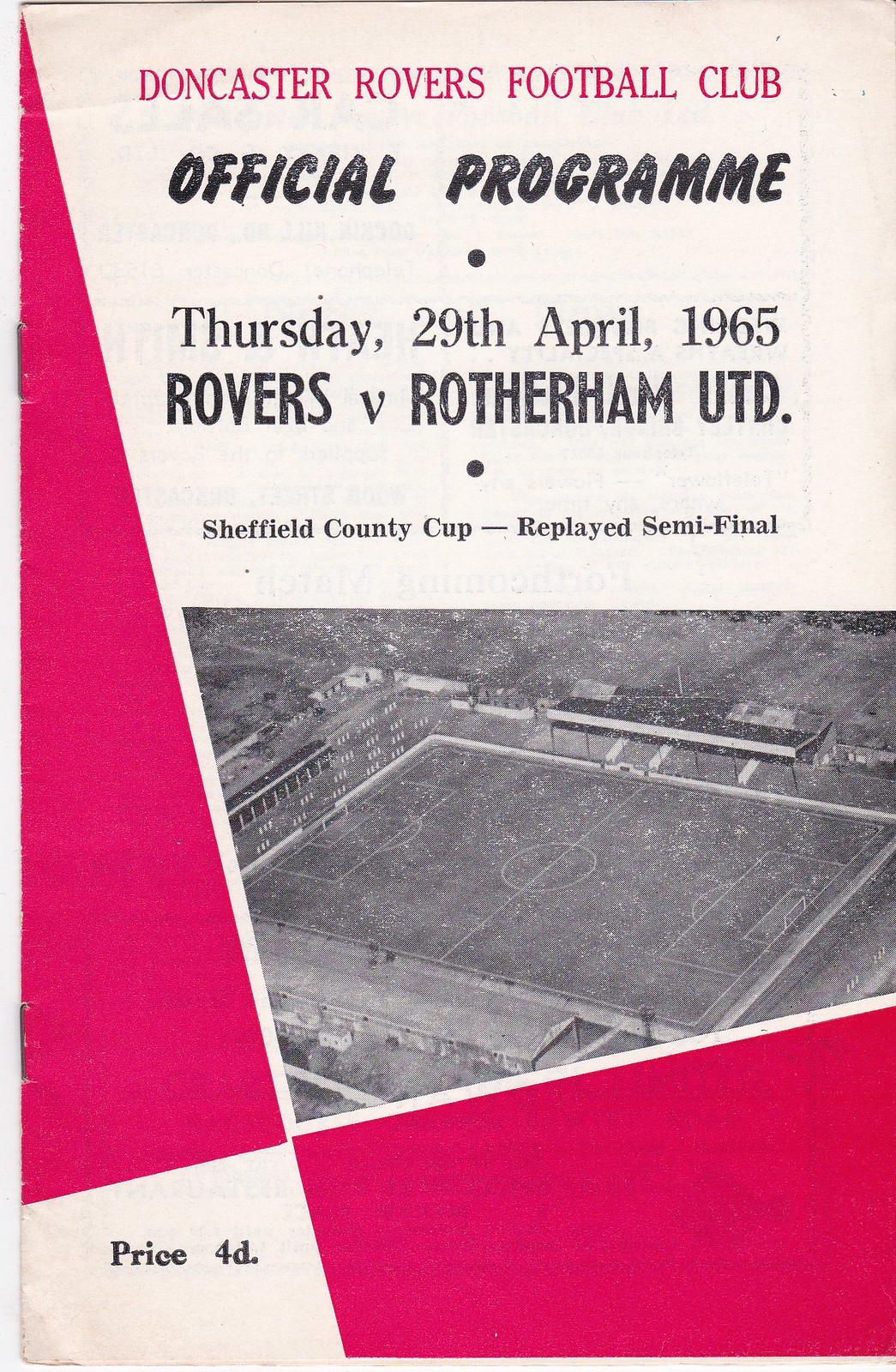This image is the cover of a vintage football program for the Doncaster Rovers Football Club, dated Thursday, 29th April 1965. The cover features a distinctive white and red design with a mildly tilted large checker pattern comprising four panels. At the top, in bold red letters, it reads "Doncaster Rovers Football Club." Directly beneath this, in black text, it states "Official Program." The program details the Sheffield County Cup Replayed Semi-Final match between "Rovers vs. Rotherham UTD." Moreover, an overhead black-and-white photograph of a football field is set within a trapezoid frame in the center of a larger white square. This grainy and low-quality image shows the entire pitch, including the stands on the sides. Surrounding the photograph are red graphic elements on the left and lower right. In the bottom left corner of the cover, the price is marked in black print as "Price 4D."